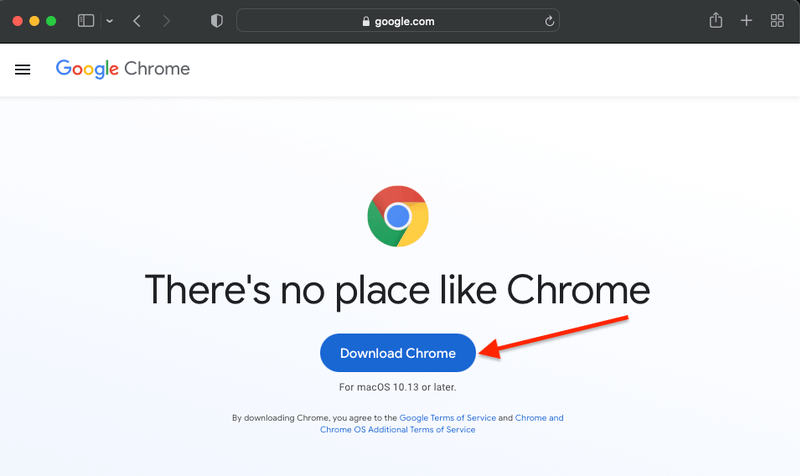The image depicts a web browser interface featuring a black border at the top. On the left side of this border, there are three circles in a horizontal line: a red circle, a yellow circle, and a green circle, representing the typical close, minimize, and maximize buttons. Additionally, there are back and forward navigation buttons.

Below the top border, there's an address bar displaying the URL "google.com" with a lock symbol indicating a secure site. Adjacent to it, a refresh button is visible. Also present is a forward icon paired with a plus symbol. To the right, there are four small squares arranged in a grid to form a larger square, likely representing a tab or window management option.

The main section beneath the address bar features a white background with a prominent hamburger menu (three stacked lines) in the top left corner. Adjacent to this menu, "Google Chrome" is written in the iconic, multicolored Google font. Beneath this, a light gray horizontal line spans the width of the section, and directly below is the round Google icon centered on the page.

Below the Google icon, large text reads "There's no place like Chrome." Towards the bottom of the image, a dark blue oblong button labeled "Download Chrome" is prominently displayed with a red arrow pointing towards it. The text beneath the button specifies that it is for "Mac OS 10.13 or higher." At the very bottom of the image, there are links labeled "Privacy" and "Terms."